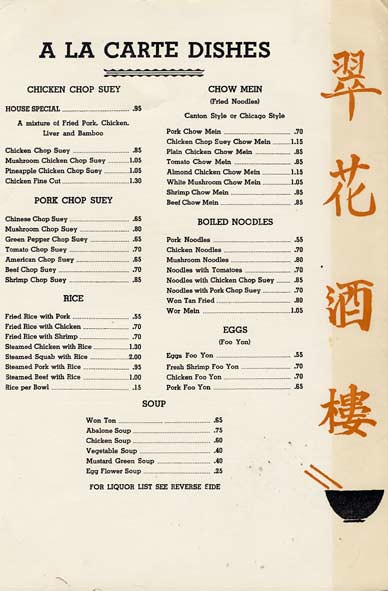This image features a restaurant menu set against a creamy colored paper background. On the right-hand side, a narrow, light tan banner extends vertically, displaying four Asian characters in a darker tan shade from top to bottom. Below these characters in the bottom right corner, there is a black rice bowl with two tan chopsticks protruding from its left side.

The menu text is printed in black and begins with a title "A La Carte Dishes," separated by an ornate squiggly line design. The menu is organized into distinct categories spread across two columns. The left column lists various options for chicken chop suey, pork chop suey, and different kinds of rice dishes. The right column offers a range of chow mein options, boiled noodles, and four types of egg dishes. Centered at the bottom of these two columns, the menu details six different kinds of soups.

At the very bottom of the menu, a note mentions beverages under the section "For Liquors, List C Beverage," although this text is somewhat difficult to read.

The careful organization and detailed descriptions reflect a variety of traditional dishes available to customers.